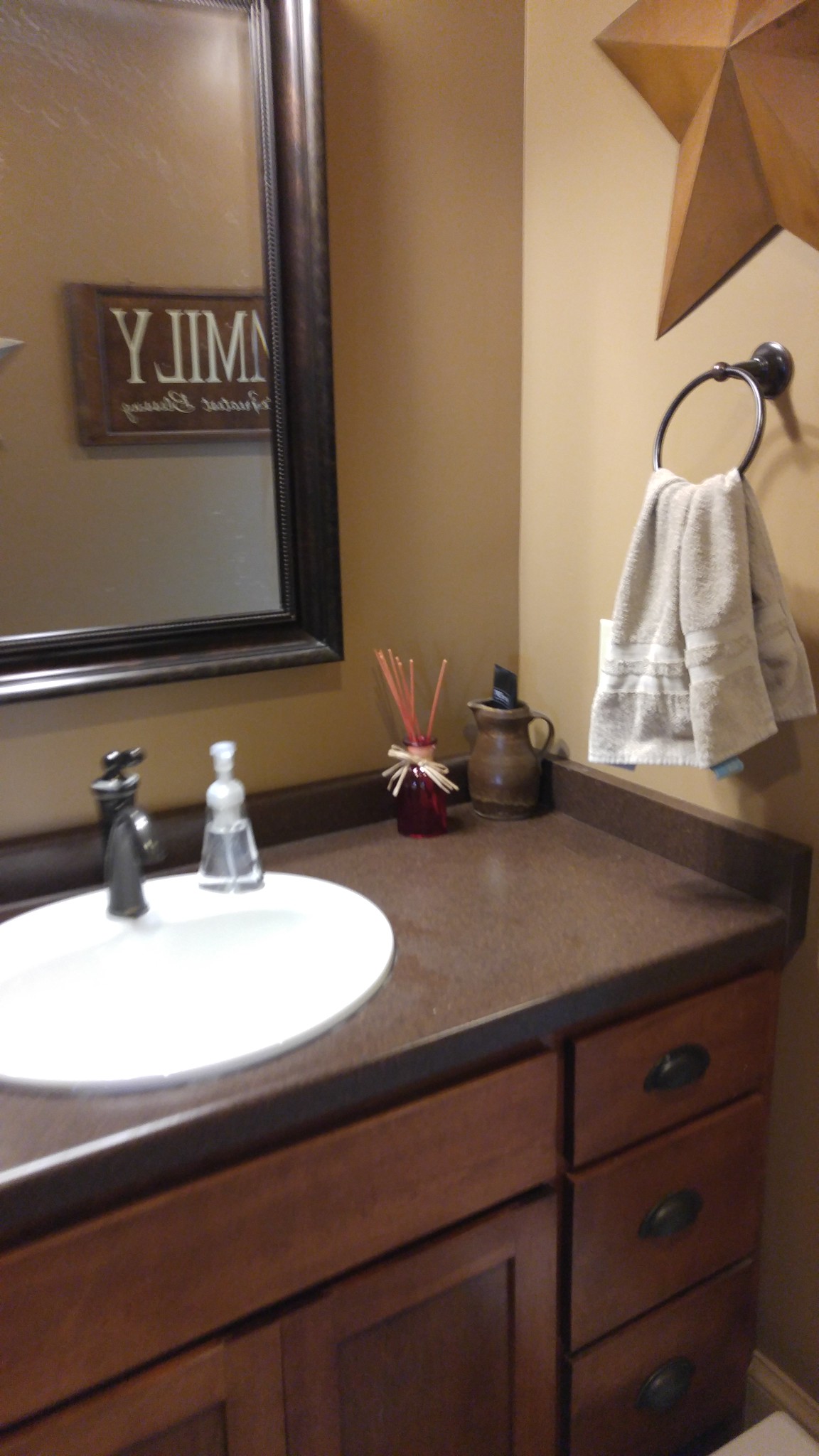This vertical color photograph captures the sink area of a cozy bathroom. The centerpiece is a pristine white sink resting atop a warm brown countertop, supported by a wooden base in a matching brown hue. This base includes three drawers and two cabinet doors for ample storage. Above the sink, a rectangular mirror with a black, picture frame-like border adds a touch of elegance. To the right of the sink, on the beige wall, hangs a round towel holder adorned with a light beige, off-white hand towel. Adding a unique decorative element, a large, star-shaped ornament in an orange hue is prominently displayed on the wall. In the reflection within the mirror, a sign on the opposite wall is visible; although reversed, it likely spells out the word "family," contributing to the bathroom's warm and welcoming atmosphere.